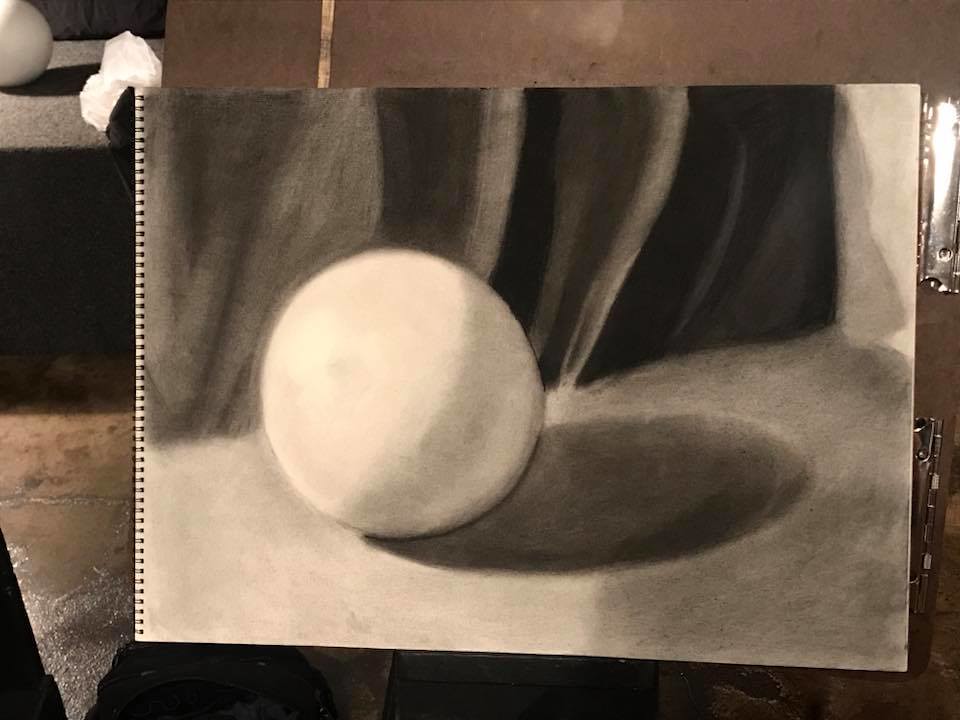This detailed photograph captures a meticulously drawn artwork on a large, artist's notebook, which features a thin black wire binding along its far edge. The notebook is set against a textured brown background, complemented by a snippet of gray fabric visible on the left and brown flooring below. The artwork itself prominently showcases a white, spherical object resting on a gray surface. The sphere casts a well-defined shadow onto the ground, contributing to the depth and realism of the drawing. The background consists of gray ripples, adding a subtle dynamic effect that contrasts with the simplicity of the central white sphere.